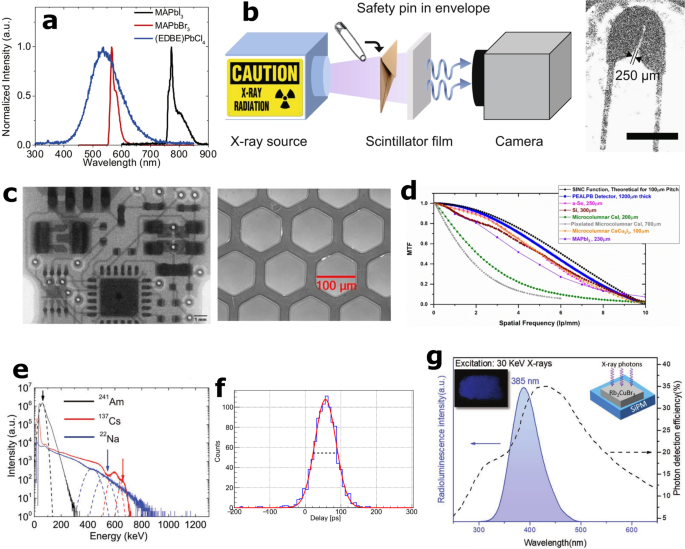The composite image consists of seven labeled diagrams (A-G) depicting various scientific measurements and schematics. Diagram A, positioned at the top left, is a graph plotting wavelength (300 to 900 nm) on the x-axis and normalized intensity (A.U.) on the y-axis, featuring three curves: a blue (EDBE), a red, and a black (both labeled MAPBL). Diagram B, adjacent to A, is a detailed schematic showing an X-ray imaging setup, including an X-ray source directing radiation towards a scintillator film, a whiteboard square, and a camera aimed at capturing the resultant image of a safety pin within an envelope, labeled "Safety Pin in Envelope," with a feature noted at 250 micrometers. The following rows include various other diagrams: diagram C highlights microscopic images of a circuit and a honeycomb structure with hexagonal cells approximately 100 micrometers in length. Diagrams E, F, and D further present additional graphs and measurements related to the scientific study. Overall, the entire image provides an intricate overview of experimental setups, microscopic imaging, and graphical data representations related to X-ray technology and microscopic structures.